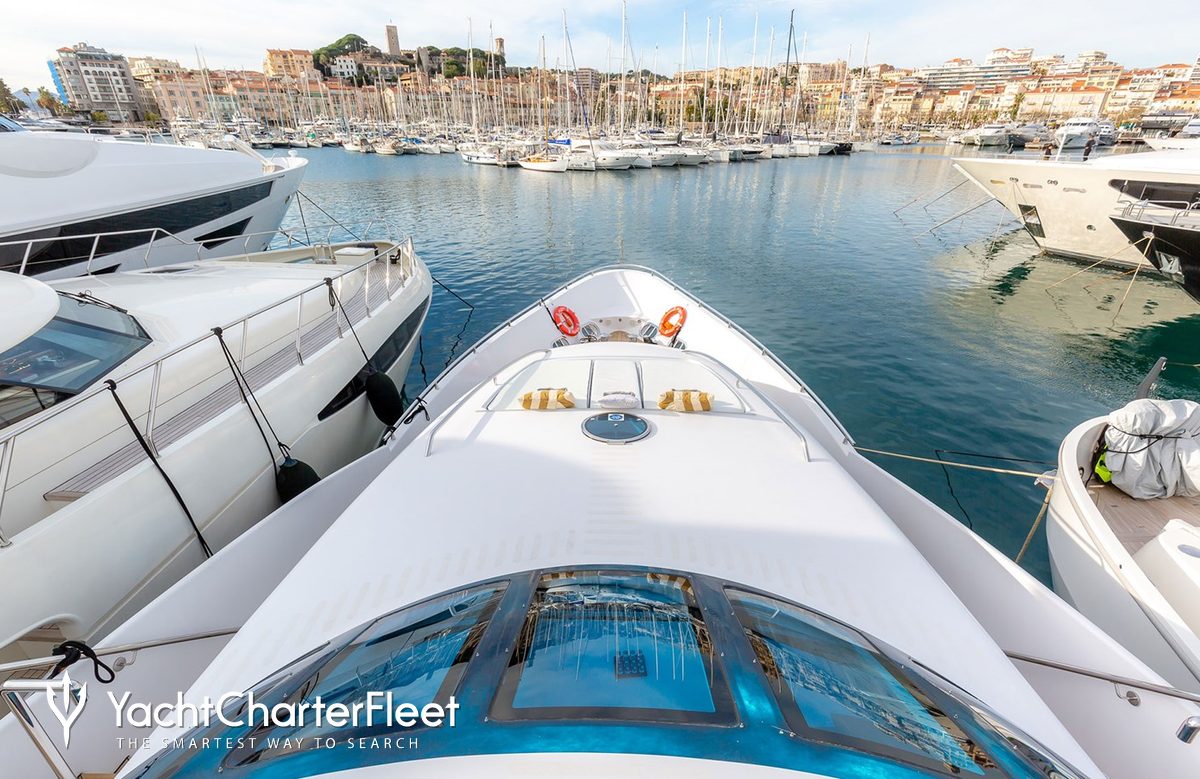This photograph captures a bustling docking area, likely a harbor, filled with numerous boats and yachts. The scene is lively with a variety of vessels, all primarily white, clustered together like a boat parking lot. Prominently in the foreground, there are four boats, with one central white boat featuring blue glass panels, possibly a see-through bottom, and displaying a couple of orange and pink life rings. The lower left corner, in white letters, reads "yacht charter fleet," followed by "The smartest way to search" in capital letters.

In the background, a mix of light yellow and orange buildings line the waterfront, extending across the image from left to right. Among these buildings are tall chimneys and a metropolitan array of both tall and short structures, suggesting a vibrant coastal city or town. There's a hill with some trees visible behind the buildings, adding a touch of greenery to the urban backdrop. 

The sky above is partly cloudy, with hues of white and blue, complementing the blue water below. The colors in the image include white, blue, orange, pink, brown, tan, and hints of light green. Despite the density and activity suggested by the boats, there are no people visible in the image. The overall composition beautifully balances the natural elements with the bustling harbor life.